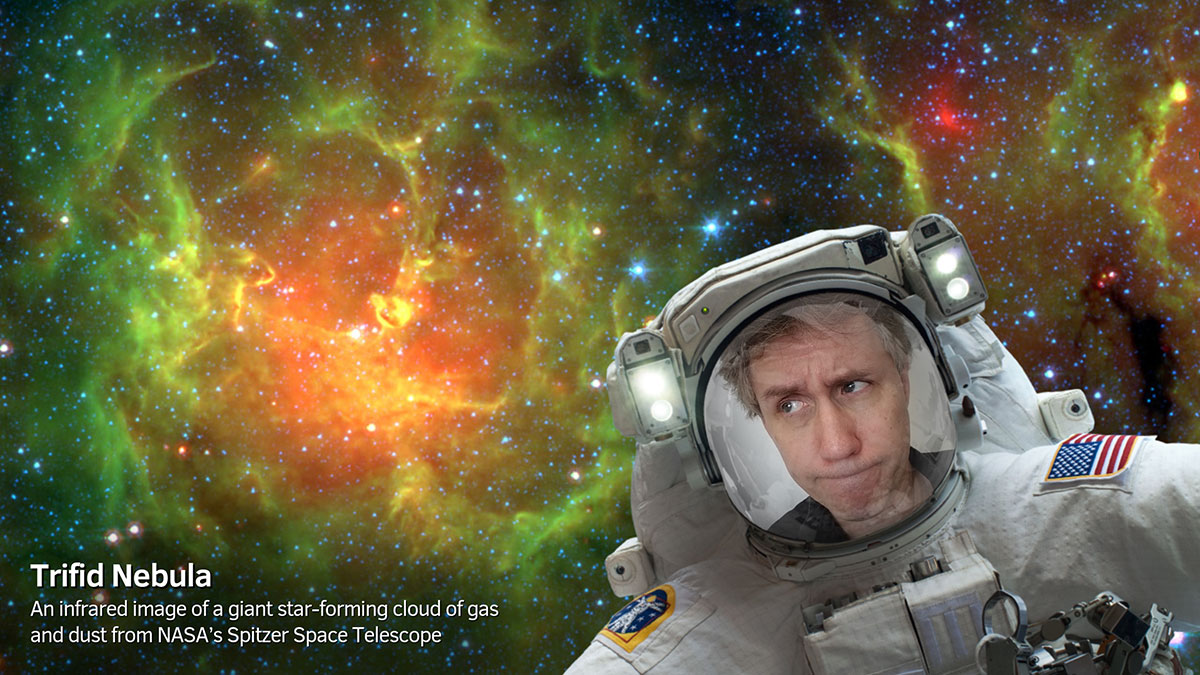The image showcases a stunning space scene with a swirling display of green and orange hues, reminiscent of a galaxy or wormhole, against a backdrop filled with white, blue, and red stars, as well as dark, cloud-like structures. Positioned prominently in the bottom left, a Caucasian astronaut in a white NASA suit is visible from the shoulders up. The astronaut, who has short blonde hair and is making a quizzical expression, is clearly seen through the faceplate of the helmet, which is equipped with two headlights. An American flag patch adorns the astronaut's left shoulder. Text in the bottom left corner identifies the scene as the "Trifid Nebula," followed by a caption that reads, "an infrared image of a giant star forming cloud of gas and dust from NASA's Spitzer Space Telescope." The overall composition of the image is an intricate blend of celestial elements and vivid colors, creating a mesmerizing portrayal of space.